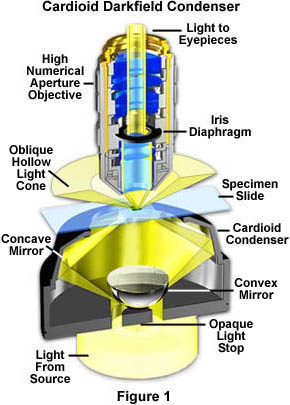The image is a detailed scientific diagram of a cardioid darkfield condenser, showcasing the intricacies of this optical equipment. The diagram, presented as a cross-sectional view to reveal the internal components, is labeled with several key parts. Notably, it includes the high numerical aperture objective, iris diaphragm, and light to eyepieces, allowing precise optical adjustments. The cardioid condenser, critical for darkfield microscopy, is prominently featured alongside a concave mirror and a convex mirror, which help in focusing and directing light. 

Additionally, the oblique hollow light cone and an opaque light stop are illustrated, essential for manipulating light paths. The diagram also displays the specimen slide where samples are placed for observation. The color scheme is varied, with significant components highlighted in blue, yellow, gold, black, white, and light blue for visual distinction. There's a yellow base labeled "light from source," indicating the origin of illumination. The text "Figure 1" at the bottom identifies the diagram systematically.

Overall, it's a comprehensive depiction of a cardioid darkfield condenser, emphasizing its functionality and componentry in a visually detailed and informative manner.